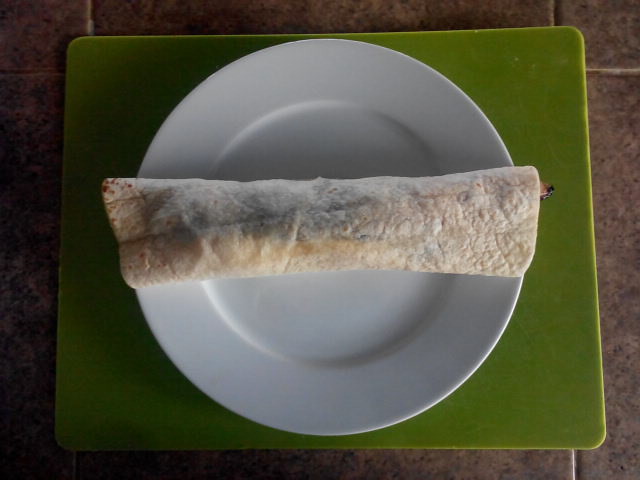This detailed image depicts a burrito placed horizontally on a perfectly round white plate. The white plate is set on a light lime green, rectangular mat with soft corners, which lies atop a brown, tiled counter, possibly kitchen flooring. The burrito itself is a typical off-white, beige color, and a piece of chicken slightly protrudes from its right side. Notably, the left end of the burrito extends just beyond the perimeter of the plate by about an inch. The lighting creates a gradient effect, with the left side of the photo being darker than the right, accentuating the contrasting textures and colors of the culinary setup.